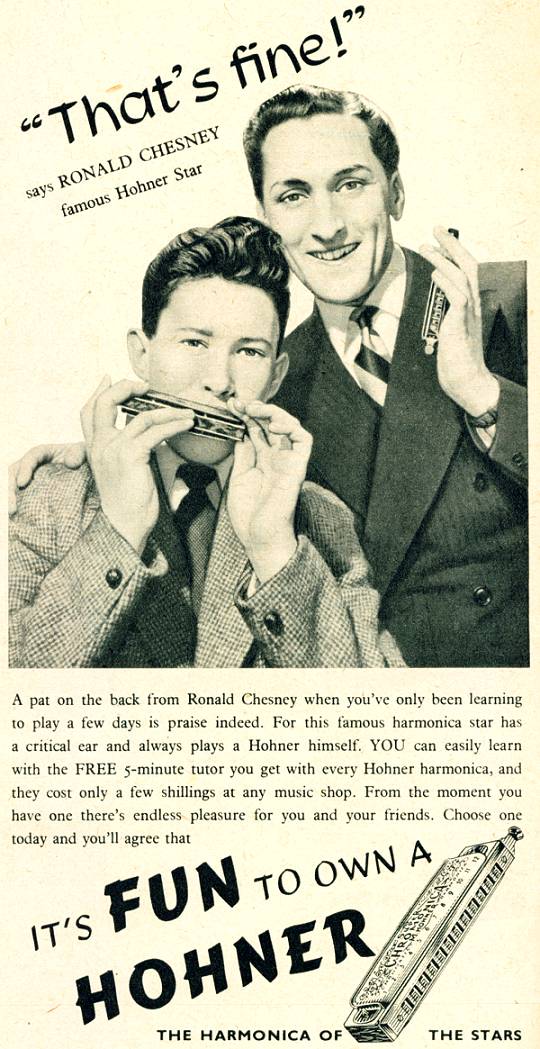This image, resembling an old newspaper or flyer, features a vertically aligned rectangular layout with a nostalgic, slightly yellowed appearance. At the top, bold diagonal print in quotation marks reads, "That's fine!" attributed to Ronald Chesney, noted as a famous Hohner star. Below this text, a black and white photograph showcases two men, seemingly from the 1960s. One man stands on the left, playing a harmonica, dressed in a button-down jacket, a necktie, and a white button-down shirt. Beside him, another man, also dressed in a suit and tie, places his right hand on the harmonica player's shoulder, holding a harmonica in his left hand.

A justified paragraph of text under the photograph offers a detailed praise-filled narrative about Ronald Chesney's endorsement of the Hohner harmonica. Following this, larger diagonal print proclaims, "It's fun to own a Hohner," with the words "fun" and "Hohner" in bold black letters. An illustration of a harmonica is displayed below this caption, and at the very bottom, the text reads, "the harmonica of the stars," emphasizing the harmonica's esteemed status. The overall design and typography suggest it's an effort to attract interest in harmonicas, promising ease of learning and an accompanying free five-minute tutor with every purchase.